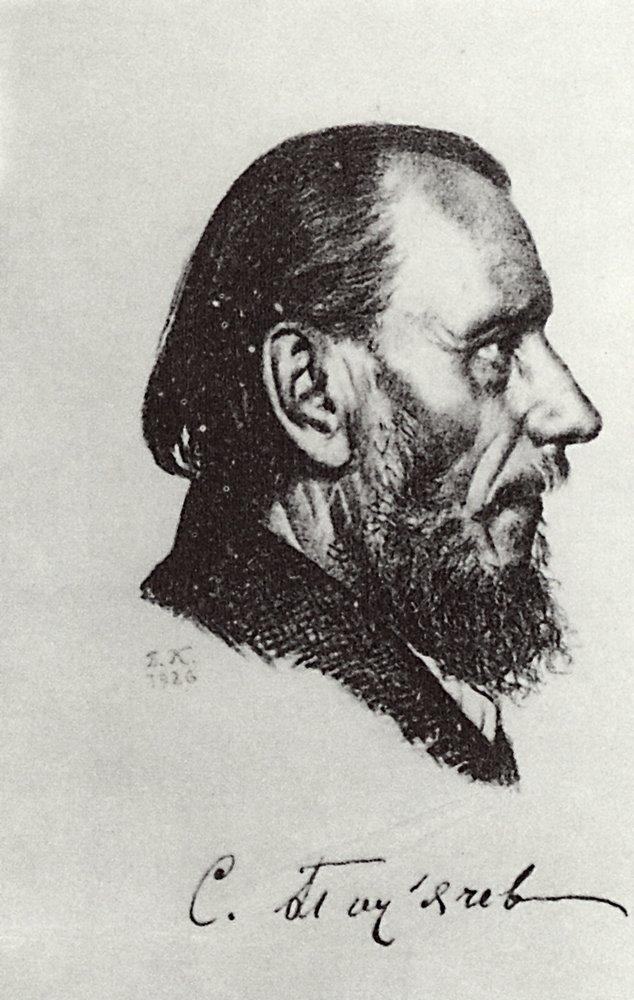The image is a detailed black-and-white ink drawing of a middle-aged to older white man, rendered on a gray piece of paper. The man is depicted in the right side profile, his gaze fixed straight ahead. His hair is slicked back and dark, with a receding hairline forming a widow's peak. The hair is slightly longer at the back, just touching the collar of his dark suit jacket. He sports a full but slightly scraggly beard that links to his sideburns, along with a mustache resting low over his upper lip. His facial features include a high forehead, a straight nose with a minor bump, and visible lower lip. The portrait includes his neck and a portion of his clothing, specifically highlighting the neckline of the jacket and a white shirt underneath. Below the bust, there's a signature in black ink, possibly reading "C.S.T.R.A.Y.S.R.E.B." accompanied by the initials "Z.K. 1926." The composition style reflects early 20th-century sketching techniques, reminiscent of turn-of-the-century Russian art, and the entire artwork is presented without a background, emphasizing the stark, precise lines of the subject against the plain parchment-like surface.